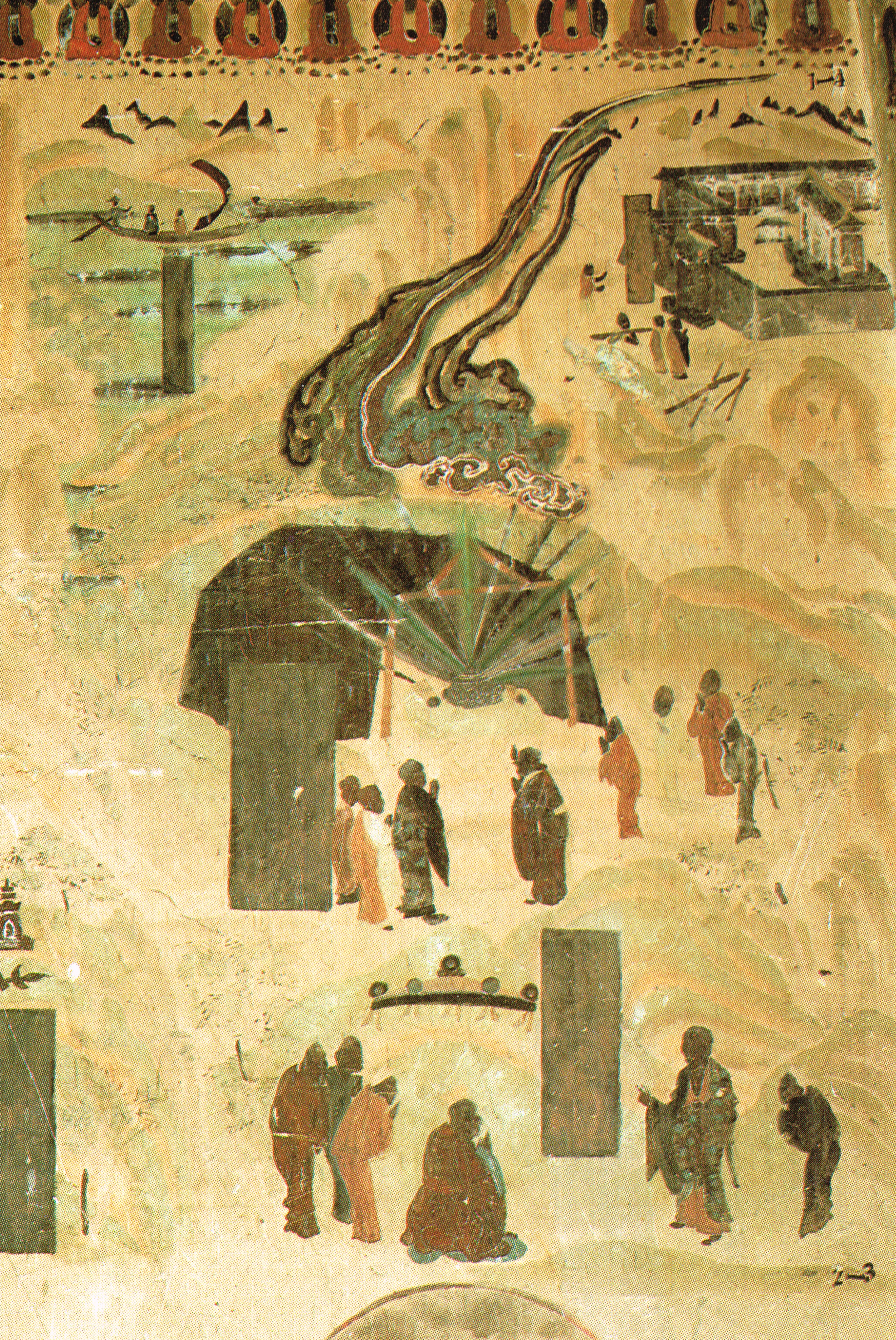The image appears to be a detailed hand-drawn illustration with an old, cave art or temple fresco style. At the bottom of the drawing, people are depicted, some sitting and praying, while others are gathered. Above these figures, there's a central scene featuring more people in a tent-like structure with a green light emanating from it, their hands raised in reverence. In the center of the image, a person sits at a large table surrounded by four others, with additional figures positioned around doors and looking on. Towards the top, the illustration includes a variety of activities: on the right, people in a city engaged in labor; to the left, figures on a boat. The uppermost section seems to show a flowing road or smoke and reddish-brown shapes resembling pillars against a black background. The backdrop of the image is an aged, yellow-gray hue, and the people are mostly dressed in darker colors, though some are wearing orange. Green structures are scattered throughout the drawing, adding to the intricate and somewhat mysterious narrative of the scene.